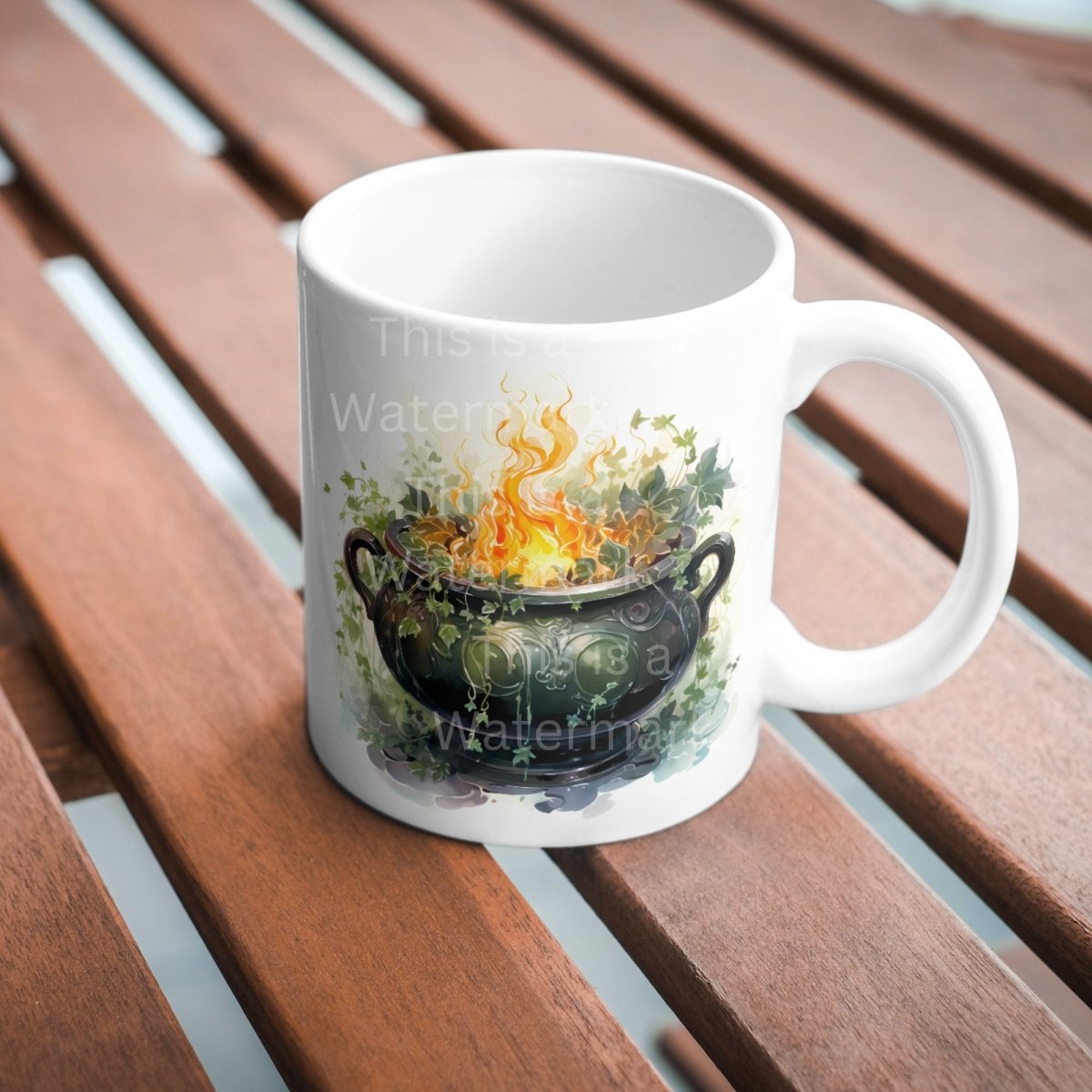This photograph captures a white coffee mug positioned on a rich, brown wooden surface composed of rectangular wooden panels with noticeable gaps between them. The mug's handle is on the right side of the image. The main design on the mug features a shiny, dark green cauldron with orange and yellow flames emanating from it, accompanied by dark green leaves at the top. Additionally, the image includes a transparent repeating watermark that reads "this is a watermark," ensuring the photo's authenticity and protecting the photographer's credit.